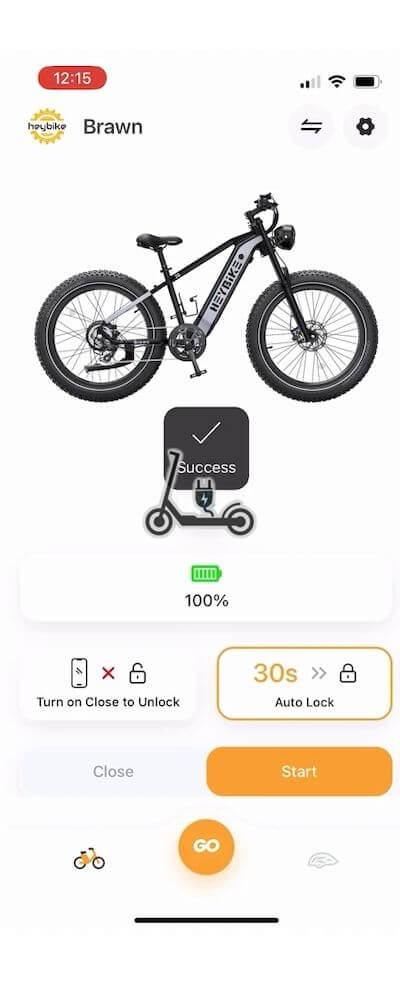**Detailed Description:**

The image is a screenshot taken on a mobile phone displaying a webpage from a website with details about a bicycle, specifically an electric bike. The webpage features a clean, white background.

**Header Section:**
- At the very top-left corner of the screen, there is a red, capsule-shaped bar showing the current time as 12:15.
- On the top-right corner, three status icons are visible:
  - A four-bar signal indicator with two of the four bars in black, indicating signal strength.
  - A Wi-Fi symbol resembling expanding light rays.
  - A battery icon showing a near-full charge.

**Logo and Page Content:**
- Directly beneath the status icons, there is a logo featuring two gold crowns and the text "hay break" in the center. Adjacent to the logo, the word "Braun" is written with two small symbols on the right:
  - One symbol is a circle with arrows facing opposite directions.
  - The other is a circle with a black gear inside.

**Main Image and Specifications:**
- The main focus of the webpage is an electric bike, prominently displayed with thick tires. This is the “hay bike.”
- Below the image of the electric bike, there is a black box with the text "Success" and an accompanying checkmark. A scooter icon with a plug plugged into the "Success" box is positioned beneath it.
- An adjacent battery icon displays a fully charged battery, indicated by a green bar and "100%."

**Navigation Boxes:**
- Below the battery indicator, there are several navigation boxes:
  - The first box on the left reads "Turn on close to unlock" and includes icons for a cellphone, an X, and a lock.
  - Next to it, there is a box labeled "30 seconds" with two arrows pointing to a lock. This box is highlighted in gold and indicates an auto-lock setting.
  - Two additional options labeled "Close" and "Start" are beneath these settings, with "Start" highlighted in mustard yellow to indicate it has been selected.

**Footer Section:**
- At the bottom of the screen, there is a navigation bar containing:
  - An icon of a yellow bike.
  - A circular "Go" button.
  - An icon resembling a wing.

This descriptive caption provides a detailed overview of the webpage content, layout, and specific elements visible on the mobile screenshot.